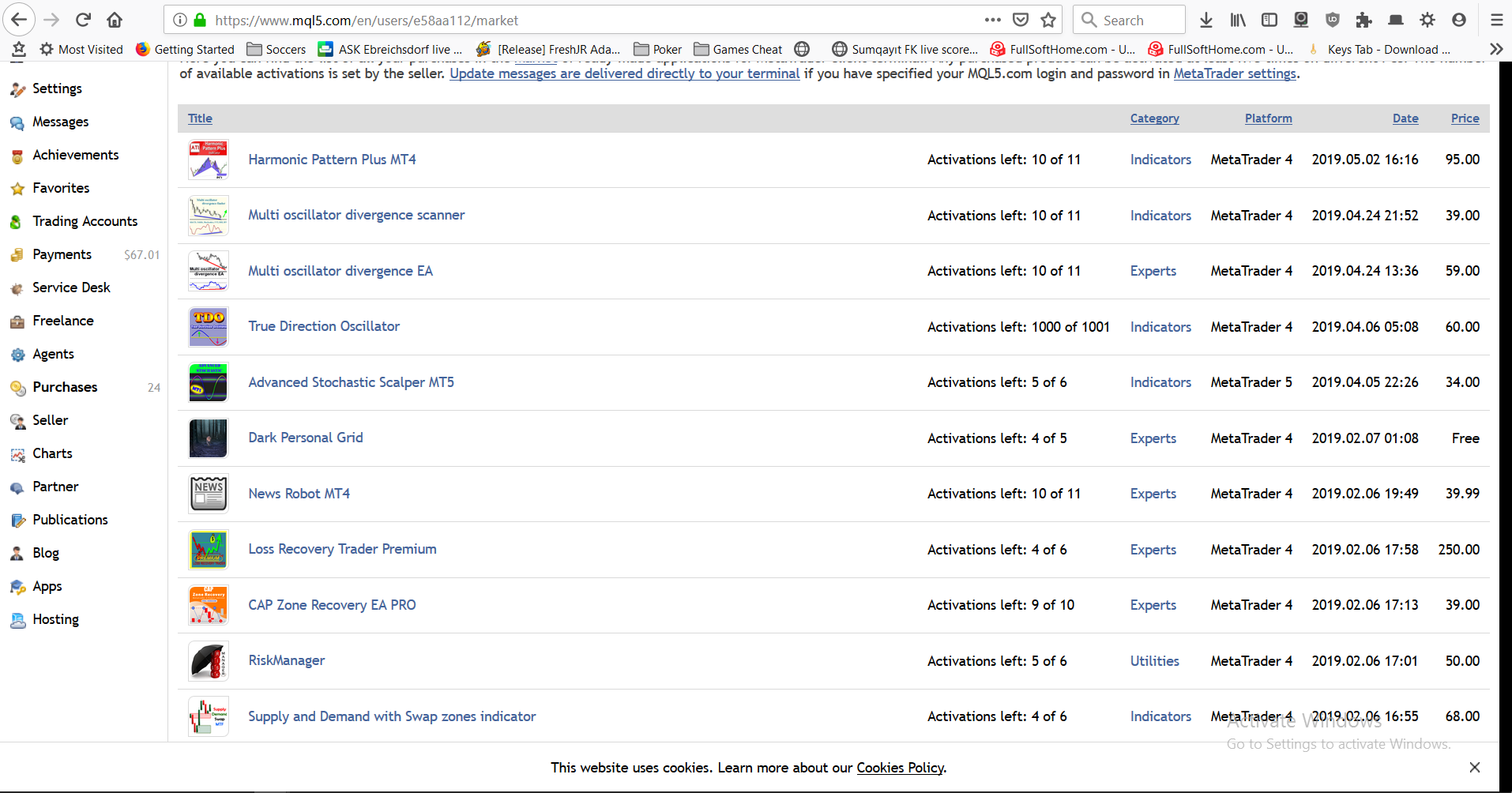A detailed webpage from MQL5.com that serves as a comprehensive resource for advanced financial trading, particularly catering to quants and algorithmic traders. The page is dense with information and somewhat challenging to read, indicative of its complex and specialized nature. The content includes various lists and categories related to sophisticated financial concepts such as oscillators, harmonic patterns, risk management, and supply and demand analysis.

The site seems to target professionals with advanced degrees in mathematics and engineering, providing tools and information for quantitative analysis and algorithmic trading. The interface includes a white background with text in blue or black, ensuring high readability of the densely packed information. On the left side of the page, there's a navigation pane with sections for Settings, Messages, Achievements, Favorites, Trading Accounts, and Agents. Various categories like Experts, Indicators, and Utilities are also visible, each likely containing a wealth of resources and tools for advanced trading strategies.